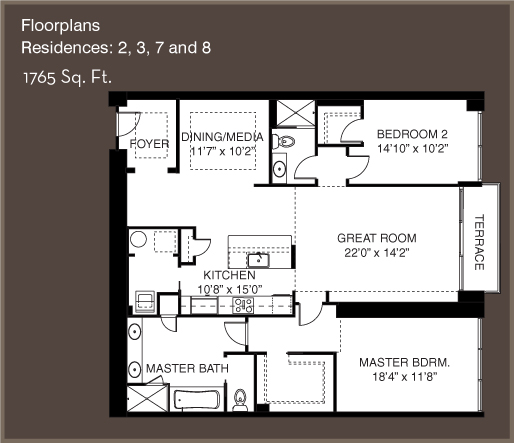This detailed and slightly horizontal floor plan image features a dark brownish-gray background, with the floor plan itself rendered in white, accented by heavy black borders and room dividers. All labeling is depicted in all-caps black ink. 

In the upper left-hand corner of the diagram, set against the dark background, the text denotes "FLOOR PLAN" along with the information "RESIDENCES 2, 3, 7, AND 8 - 1,765 SQ. FT."

The layout begins with a single door at the upper left corner, which opens into a foyer. This foyer leads seamlessly into an expansive great room that incorporates a kitchen. Behind the kitchen on the left side is a bathroom. 

Adjacent to the foyer, at the top left of the floor plan, is a designated dining/media area. In the upper right corner, Bedroom 2 is situated, complete with an attached bathroom accessible both from this bedroom and the great room. 

The great room extends to a terrace located at the center right of the plan. The lower right corner houses the master bedroom, which measures 18 feet 4 inches by 11 feet 8 inches. This master suite boasts a spacious walk-in closet and an en-suite master bathroom. 

The master bathroom features a dual-sink vanity, a shower, and a tub, all of which are encompassed within an open space for the toilet that lacks a door. 

The kitchen is designed with an island containing a sink at its center, while the primary appliances are installed along the back wall, which is shared with the master bath in the lower left corner.